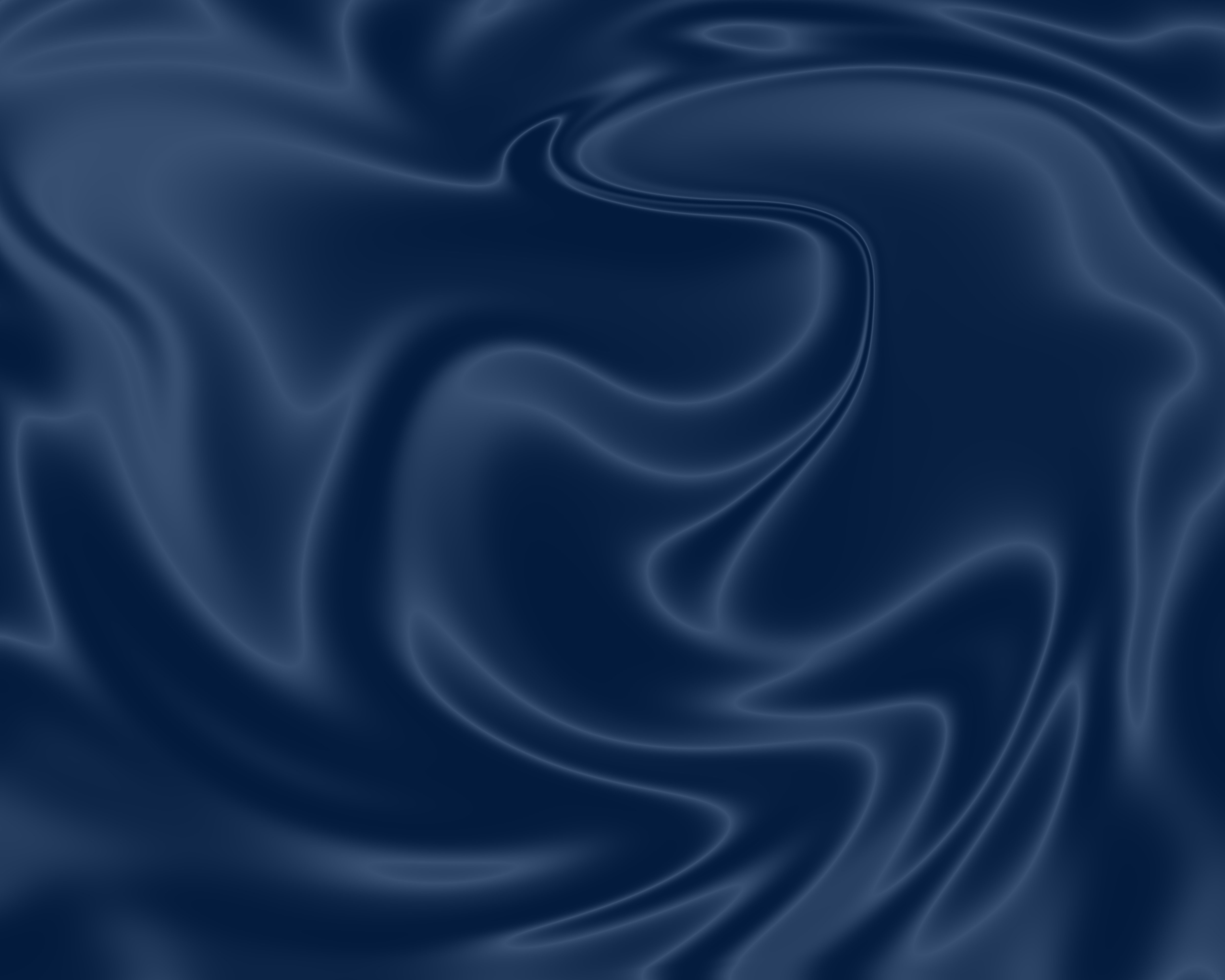The image is a slightly rectangular landscape of what appears to be a rich, silky fabric in varying shades of blue, ranging from deep navy to almost glowing white. The fabric is elegantly draped with smooth, flowing folds and contours, creating a sense of movement and light reflection. The background is entirely blue with no additional elements, people, or text. The lighter areas of the fabric seem to catch and reflect light, adding a velvety texture and an air of luxury, class, and elegance to the scene. The upper left corner contains brighter, almost white highlights, while the lower left is the darkest blue, giving depth and dimension to the fabric's smooth curves and neat curls. There are no sharp angles or borders in the image, enhancing the sense of softness and sophistication.